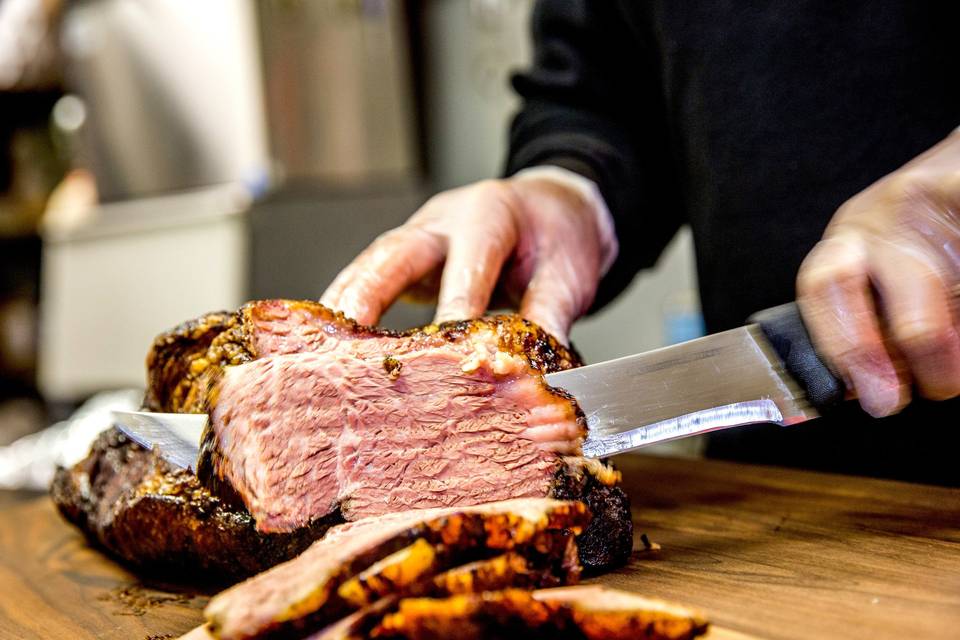In this close-up image, a man wearing a black suit jacket over a long-sleeve white shirt is meticulously slicing a large, golden brown, and juicy slab of beef on an expansive, dark walnut-colored wooden cutting board. His gloved hands, one holding the beef and the other wielding a long, sharp knife with a black handle, work in harmony as he thin-slices the meat. The image emphasizes the precision of his slicing, showcasing several previously cut, overlapping slices in the foreground. Despite the background being blurred, one can make out the indistinct form of a commercial ice machine, further directing the viewer’s attention toward the detailed textures and colors of the meat and the act of slicing in the foreground.